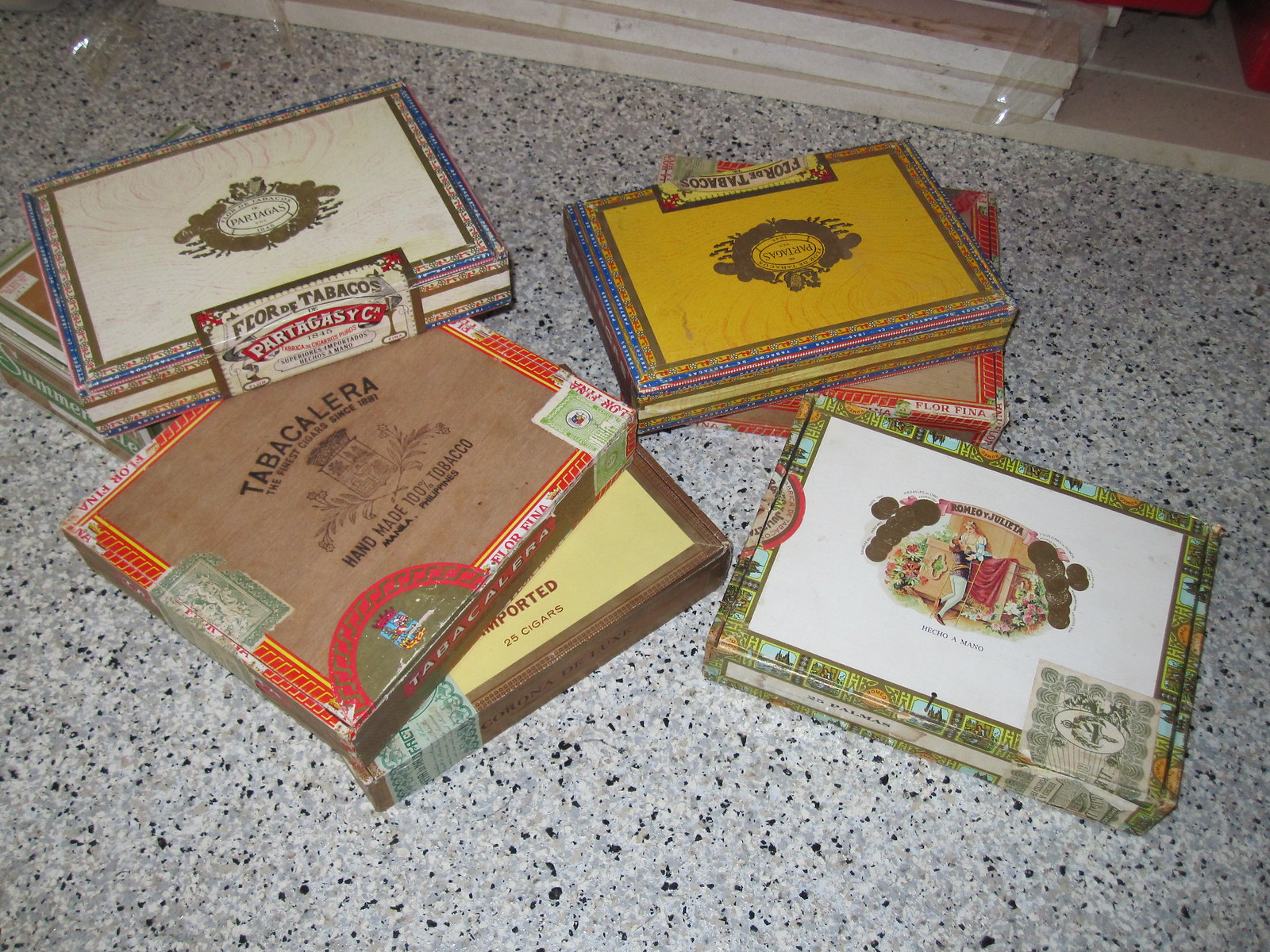The photograph is a detailed close-up of seven colorful, vintage tobacco boxes, presumably for cigars, carefully arranged on a speckled countertop that appears to be made of granite or marble, featuring a mix of white, black, gray, and green specks. The tobacco boxes, which vary in color and design, include intricate embroidery in shades such as blue, red, yellow, brown, and light brown, with one notably adorned with multicolored pictures that feature green, light blue, and orange hues. 

The prominently displayed boxes present a range of branding. One box in the forefront showcases a gold logo with a white circle labeled "PARTAGAS", while another to the right sits atop a tan and red box bearing the same logo. Yet another box is distinguished by the label "TABACALERA, the finest cigars since 1881, handmade 100% tobacco, MULUNA PHILIPPINES," with 25 cigars indicated beneath in a yellow and brown design. Another notable box carries the text "RONEO AND JULIETTE" and depicts an illustration of a woman in a blue dress and a man in a tuxedo and white pants with brown shoes. 

Adjacent to the tobacco boxes are stacks of light brown wood, partially wrapped in plastic, adding a rustic element to the scene. The photograph, captured in color, seems to suggest these could be either newly purchased or items intended for sale, highlighting the diversity and vintage charm of the cigar boxes.